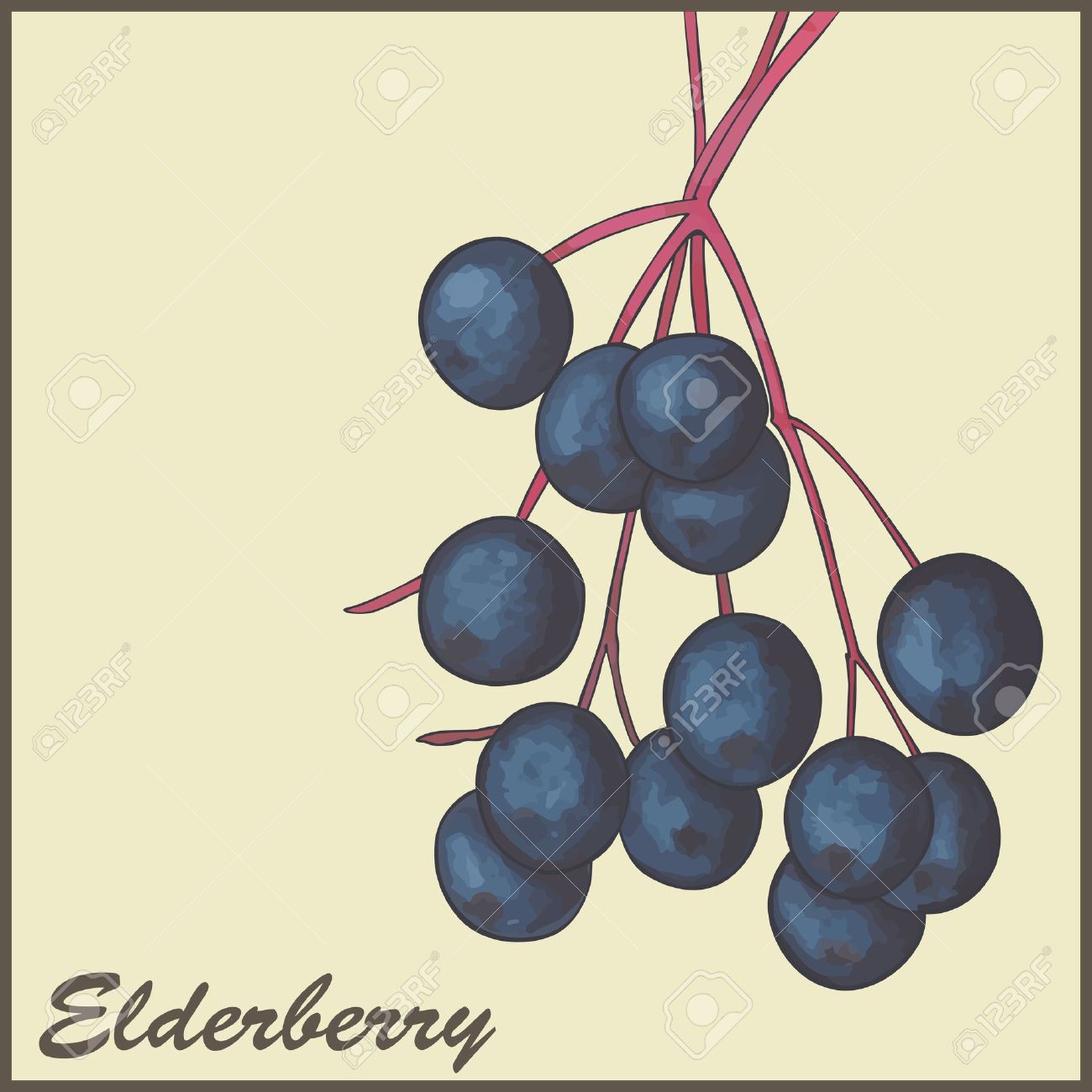This detailed image presents a cartoonish-style drawing of elderberries on a reddish-pink vine. The vine, which traverses from the top and branches out into multiple smaller stems, holds a cluster of dark blue-purple elderberries, totaling approximately 10-13 berries. These berries resemble blueberries but are clearly identified as elderberries by the cursive text "elderberry" inscribed in brown in the bottom left corner of the square image. Encasing the light yellow background, which contrasts nicely with the vine and berries, is a brown-colored border. The image also bears watermarks, including small camera icons and the text "123RF," with light crosses overlaying the artistic depiction.